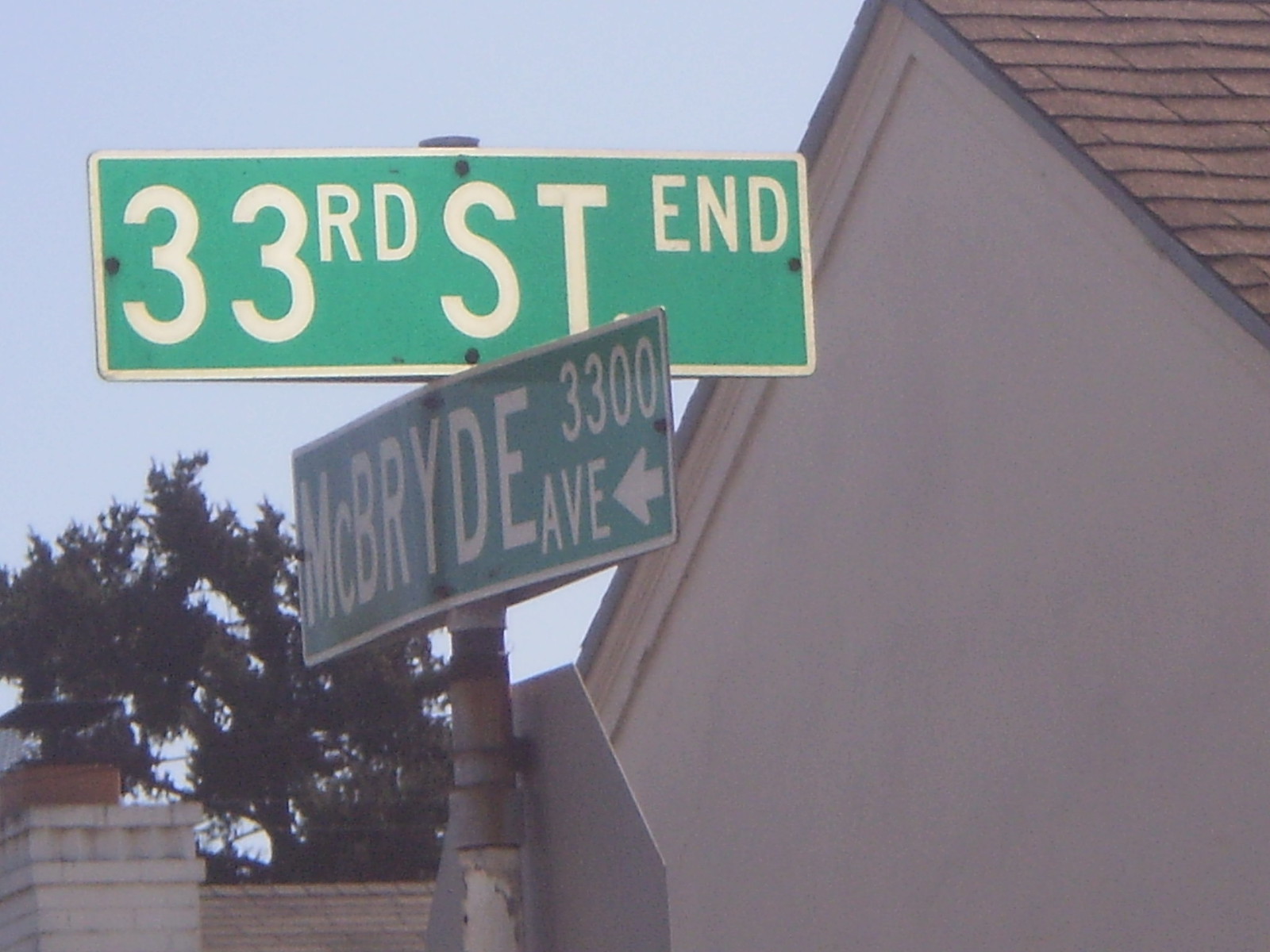This photograph captures an intersection marked by two aged and slightly dirty green street signs with white text. The top sign reads "33rd Street End" and the one below it indicates "McBride Avenue 3300." Both signs are mounted on a silver metal pole, which also holds a stop sign, visible only from the back with its characteristic octagonal shape. The signs are positioned on the left side of the image, occupying the top left corner. The scene is set in a neighborhood, with a tan or off-white house featuring brown roof shingles and part of a white brick wall visible in the background. Additionally, a chimney and a tree with leaves against a blue sky add to the backdrop. The side of another house, possibly tan, appears on the right side of the frame, contributing to the detailed yet mundane neighborhood scene.